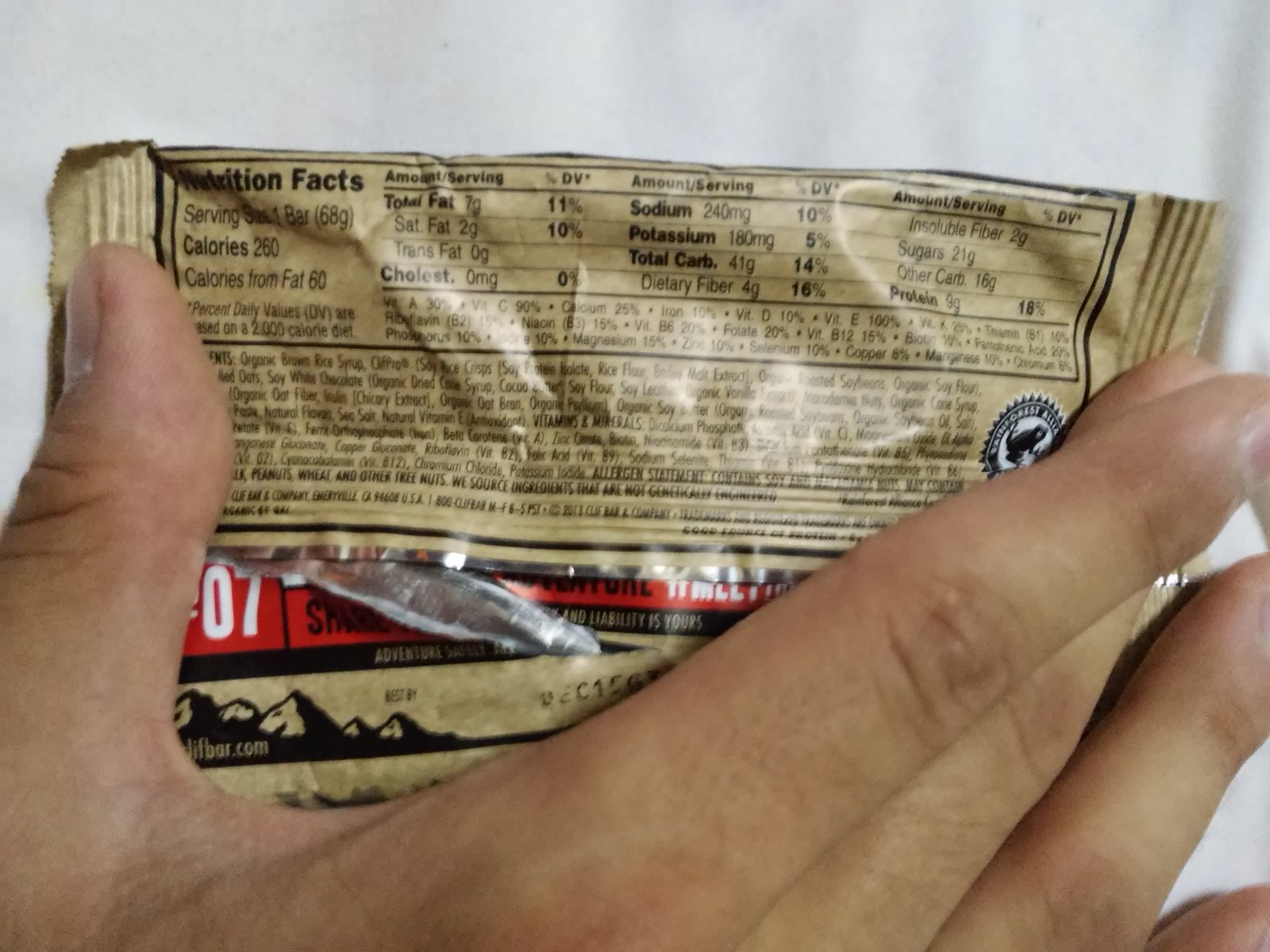A detailed top-down view of an empty khaki-colored plastic packaging is displayed on a white sheet background. The packaging, shown from the back, is stretched flat by a hand, revealing where it is torn on the inside. The nutritional facts label dominates the top half of the packaging, printed in black ink and providing extensive nutritional information. Below it, the bottom half contains a comprehensive list of ingredients.

The hand, appearing to be of a light to slightly darker skin tone, is positioned at the bottom of the image. The thumb is seen on the left side, while the other four fingers are on the right, with the pointer finger raised. The image is cropped just above the knuckles, focusing attention on the packaging.

Additionally, a small sticker-shaped symbol featuring an icon of a frog is visible on the packaging. Near the bottom, there's a red bar accompanied by a white "07" and some black text. The lower part of the packaging also includes a silhouette illustration of a mountainscape. The end of a web address, partially reading "lifbar.com," is printed along the bottom edge.